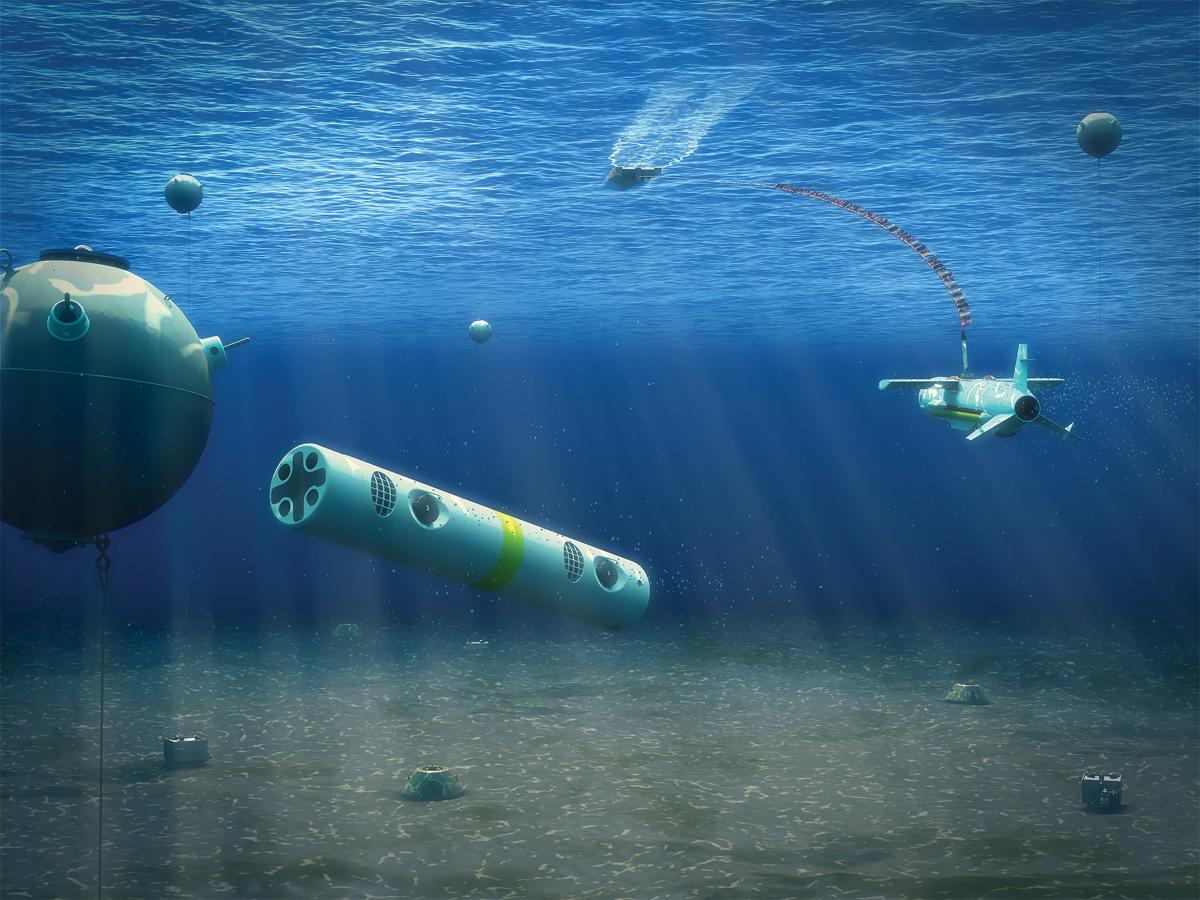An underwater scene is beautifully captured in this detailed photograph, illuminated by the gentle rays of sunlight filtering through the water from the surface. The ocean floor sprawls across the bottom of the image, scattered with various metallic fragments and machinery parts. Positioned near the center of the image is a prominent silver cylinder with a yellow stripe, floating aimlessly. To the right, a distinctive submarine with wing-like extensions and a silver strip on top hovers in the water. Three floating sea mines, or "globes," are dispersed throughout the scene: one larger and camouflage-patterned in the left center, a darker gray one above it, and another on the right. At the top of the image, the water surface is depicted with a speed boat cutting through, its white trail vividly visible. Overall, the scene combines both natural underwater elements and remnants of human activity, creating a striking and dynamic vista.